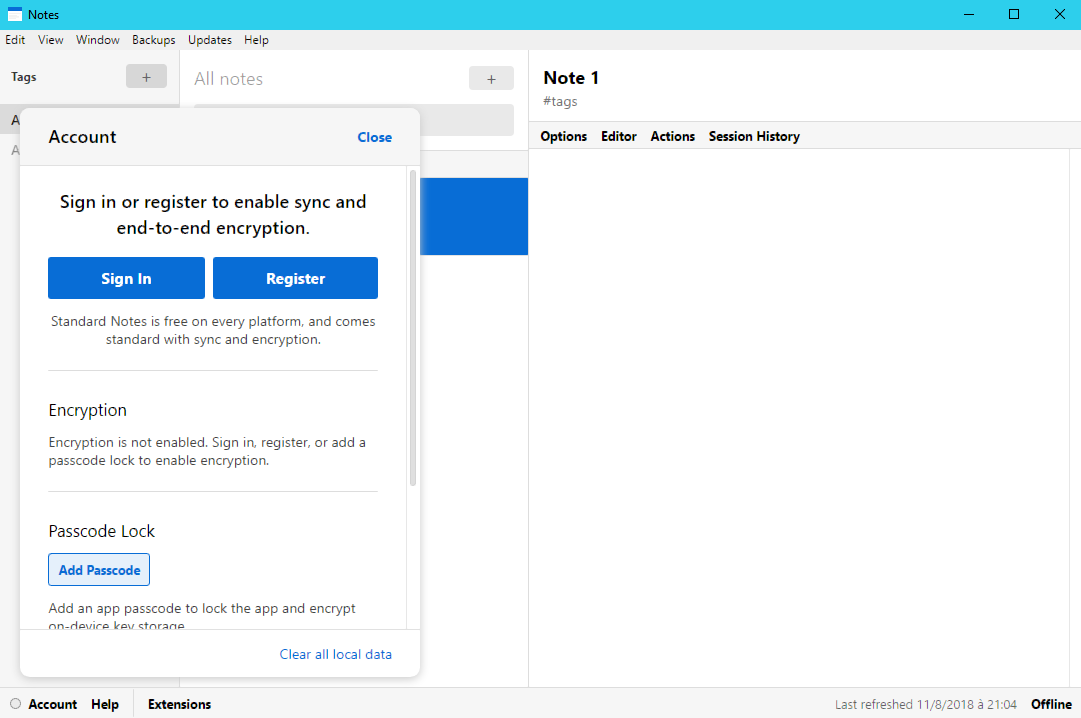The interface of a note-taking application is displayed with distinctive sections and buttons. The top section features a blue border with the label "Notes". Below this, there are menu options including "Edit," "View," "Windows," "Backup," "Update," "Help," "Tags," and "All Notes."

A prominent pop-up box with a gray border appears, titled "Account" at the top, where a blue "Close" button is also visible. Inside the box, instructions prompt users to "Sign in or Register to enable sync and end-to-end encryption," accompanied by two blue buttons labeled "Sign In" and "Register."

Further details include a statement indicating, "Standard Notes is free on every platform and comes standard with sync and encryption." Below this, a divider line separates sections, followed by text explaining, "Encryption is not enabled. Sign in, register, or add a passcode lock to enable encryption."

Continuing downward, another section labeled "Passcode Lock" includes a blue button that says "Add Passcode". It describes the function as "Add an app passcode to lock the app and encrypt device key storage." Additionally, a blue text option to "Clear All Local Data" is available.

To the right, a vertical scroll bar allows users to navigate the interface. At the bottom, options for "Account," "Help," "Extension," and "Offline" are accessible.